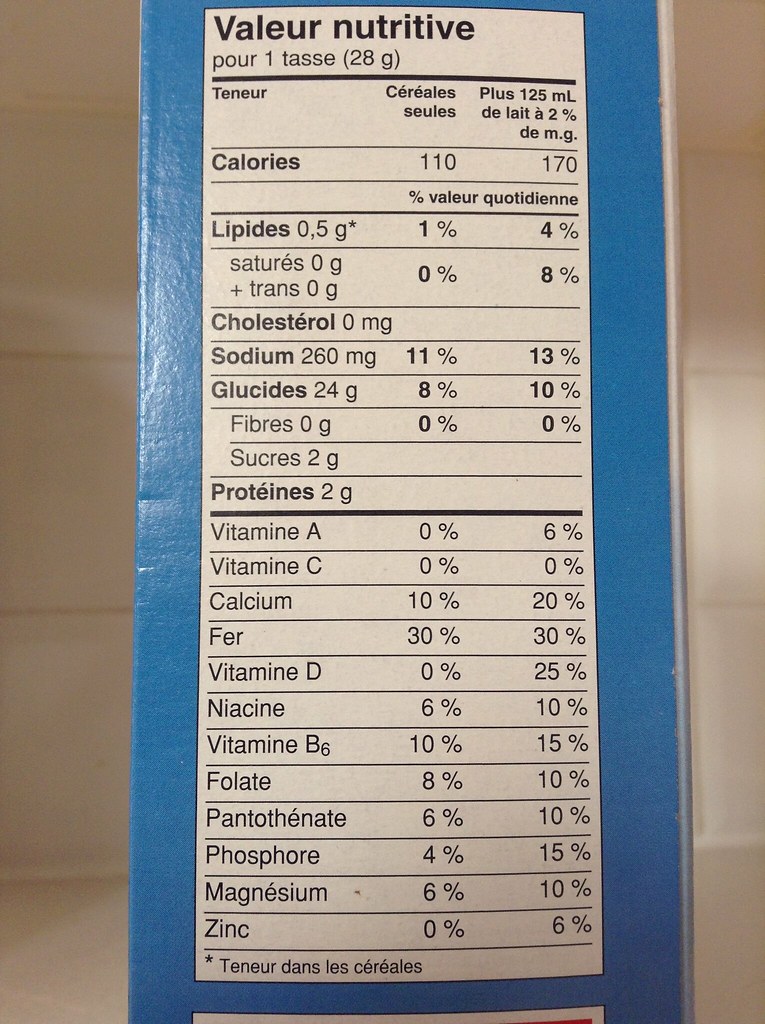A photograph of a nutrition facts label written in a non-English language. Despite the language barrier, the layout and familiar structure of the label make the information relatively easy to decipher. The label indicates the following nutritional content per serving:

- Calories: 110
- Total Fat: 0g (includes 0g saturated fat and 0g trans fat)
- Cholesterol: 0mg
- Sodium: 260mg
- Carbohydrates: Glucose 24g (Dietary Fiber: 0g, Sugars: 2g)
- Protein: 2g
- Vitamins and Minerals:
  - Vitamin A: 0%
  - Vitamin C: 0%
  - Calcium: 10%
  - Iron: 30%
  - Vitamin D: 0%
  - Niacin: 6%
  - Vitamin B6: 10%
  - Folate: 8%
  - Pantothenate (Pantothenic Acid): 6%
  - Phosphorus: 4%
  - Magnesium: 6%
  - Zinc: 0%

The label also includes additional information, but it is in a language that is not English, making it difficult to interpret further details.